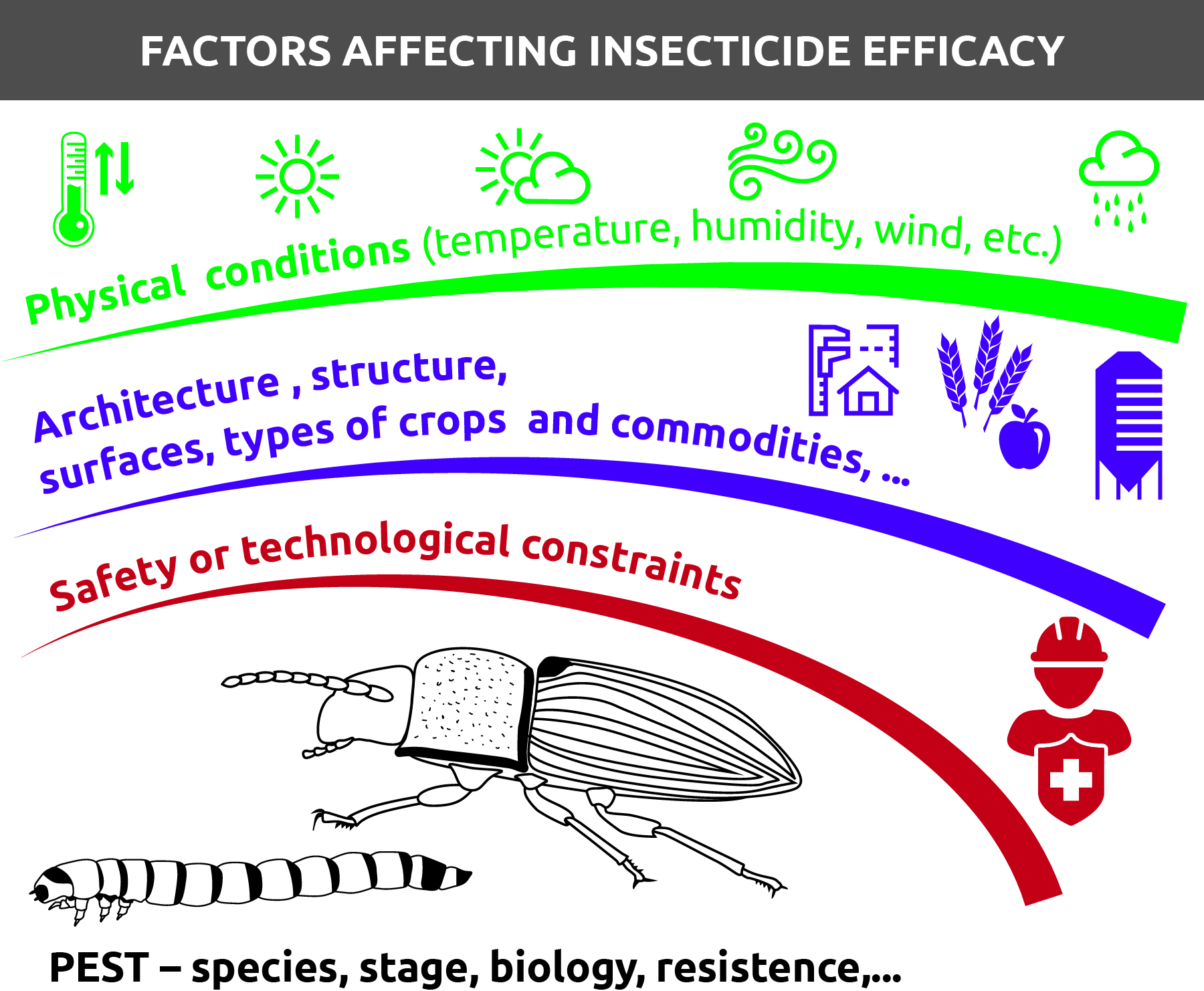This image is a public service poster on a white background with a wide gray horizontal banner at the top, featuring bold white text in all caps that reads "Factors Affecting Insecticide Efficacy." Below this header, icons and text are divided into thematic sections, each distinguished by a unique color and curved swoosh design.

The first section addresses "Physical Conditions," highlighted in bright lime green. It includes icons for various environmental factors: a thermometer (temperature), a radiant sun (sunlight), a sun partially covered by a cloud (humidity), three curving lines (wind), and a cloud with raindrops (precipitation). The green swoosh stretches horizontally across this section.

Next, the "Architectural Structure" section is in cobalt blue, emphasizing elements like surfaces, types of crops, and commodities. Blue icons include a house with a tall building, three grains of wheat accompanied by an apple, and a grain storage tower. These elements are depicted below another blue swoosh.

The third section focuses on "Safety or Technological Constraints," marked in bright red. This includes a red icon of a man wearing a hard hat or emergency responder hat and a shield bearing a white cross. This section is also separated by a red swoosh.

The final section at the bottom, in black and white, visualizes the pest factors. It shows a detailed drawing of an insect with segmented antennae and three pairs of legs, as well as a segmented larva or worm. Accompanying text in bold black letters reads "PEST - species, stage, biology, resistance."

In summary, this detailed diagram illustrates the hierarchy of various factors that impact insecticide efficacy, from environmental conditions and structural components to safety constraints and pest characteristics.